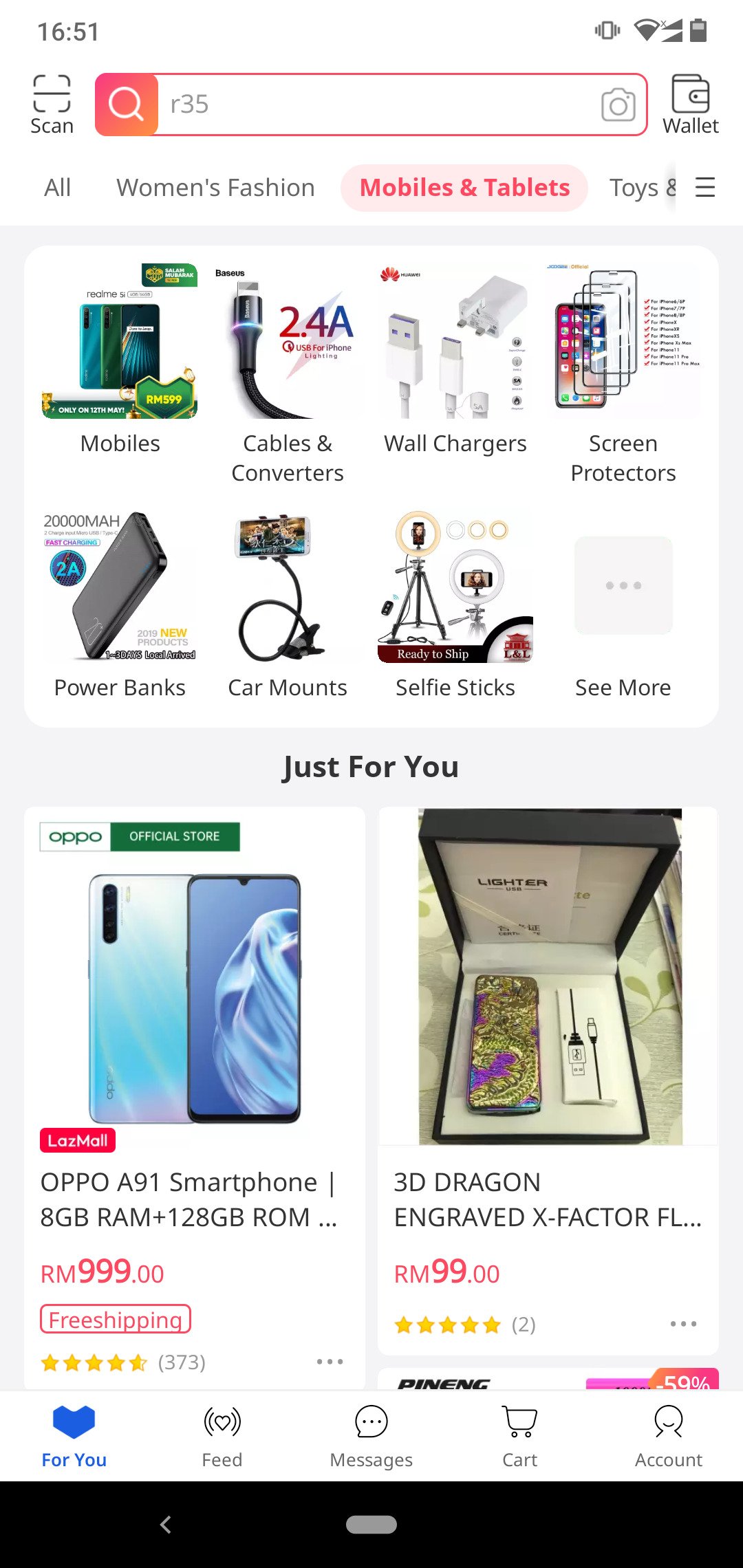The image captures a screenshot of a website tailored for shopping, taken on a mobile phone. The top of the screen indicates a time of 16:51 on the left, and on the right, various icons are visible, including a vibration symbol, Wi-Fi connection, data signal strength, and battery status.

In the search bar located at the top center of the screen, the letters "R35" have been entered. To the left of the search box, there is an option labeled "Scan," and to the right, an option labeled "Wallet." Below the search bar, a horizontal menu bar features categories such as "All," "Women's fashion," "Mobiles and tablets," and "Toys." There are more categories not fully visible in the screenshot. The "Mobiles and tablets" category is highlighted in red, set against a light pinkish background.

Descending the page, there is a series of product images and labels arranged from left to right:
1. "Mobiles" - showcasing various mobile phones.
2. "Cables and Converters" - highlighted in this section is a 2.4A USB cable for iPhone, branded by Baseus.
3. "Wall Chargers" - featuring chargers from Huawei.
4. "Screen Protectors" - though the brand name and details are unclear due to the blurriness when enlarged.

Further down, another row of products includes:
1. A "Power Bank" with a capacity of 20,000 mAh, featuring fast charging with a 2A rating displayed in a blue circle. The power bank is gray, labeled as a 2019 new product with a yellow "New" tag. It mentions shipping within one to three days locally.
2. "Car Mounts" - displaying a stand designed to hold a cell phone horizontally, secured by a clip at the bottom.
3. "Selfie Sticks" - represented by two tripod stands equipped with light rings, one pinkish and the other white, suitable for selfies or video recording. This section is labeled "Ready to ship L&L."
4. A "C-more" button is present, depicted as a gray box containing three gray dots in a horizontal line.

The "Just for You" section presents:
1. An "Oppo Official Store" product - the Oppo A91 smartphone with 8GB RAM and 128GB ROM, priced at RM999.00. It boasts free shipping, a rating of four and a half stars based on 373 reviews.
2. A 3D Dragon Engraved USB-charging lighter, referred to as the "X-Fighter," priced at RM99.00, and rated five stars from two reviews.

At the bottom of the screen, additional options include "Feed," "Messages," "Cart," and "Account," accompanied by a blue heart icon with "4U" inscribed in blue. There is no further information visible in the screenshot.